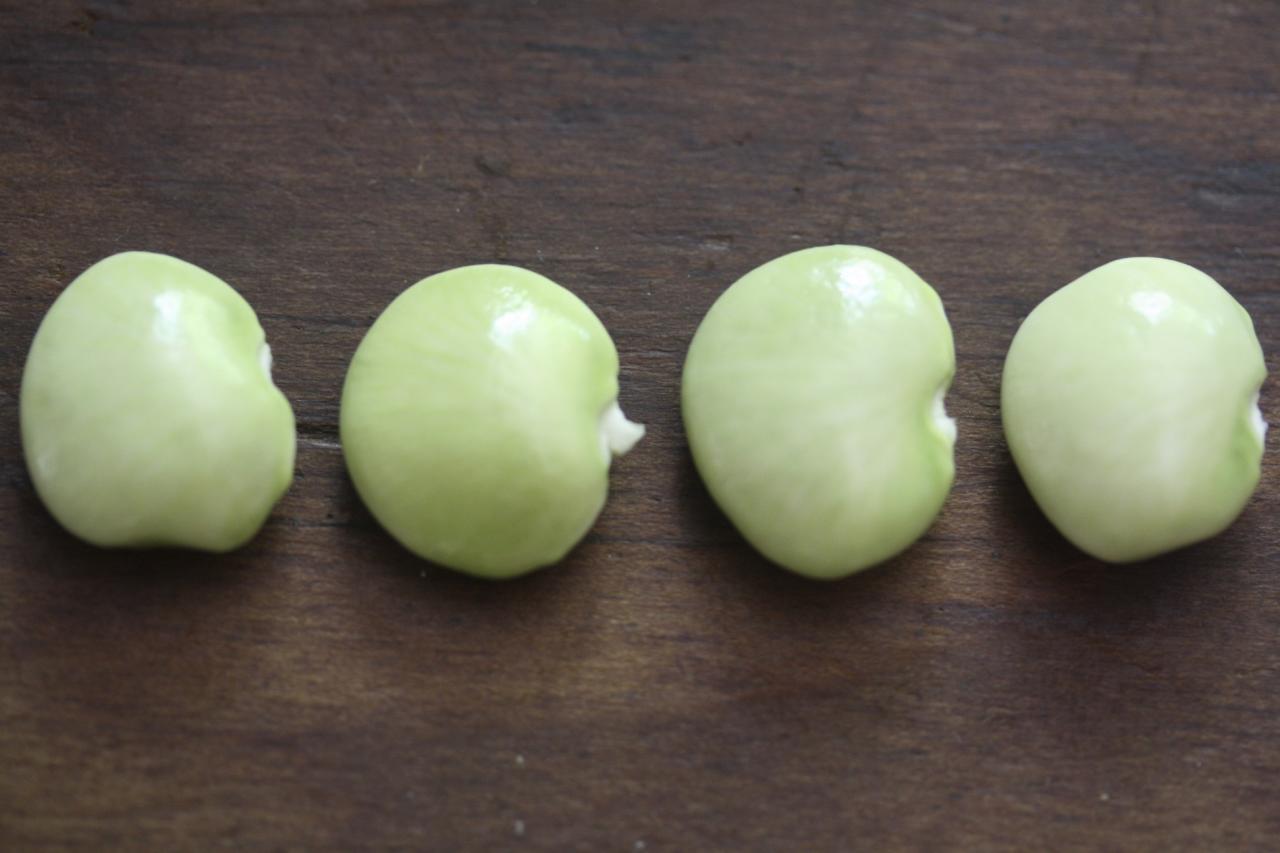This highly detailed photograph captures four plump, light green lima beans arranged in a neat row on a dark brown wooden surface. The wooden tabletop, featuring a semi-smooth grain, serves as a rustic backdrop, contrasting with the glossy beans that reflect light, creating visible white highlights. Each bean exhibits an almost circular, kidney-like shape, with a small white divot on the right side, indicative of where they were attached to their stems. The close-up nature of the image leaves no additional elements in the frame, focusing solely on the texture and simplicity of the beans and the table.